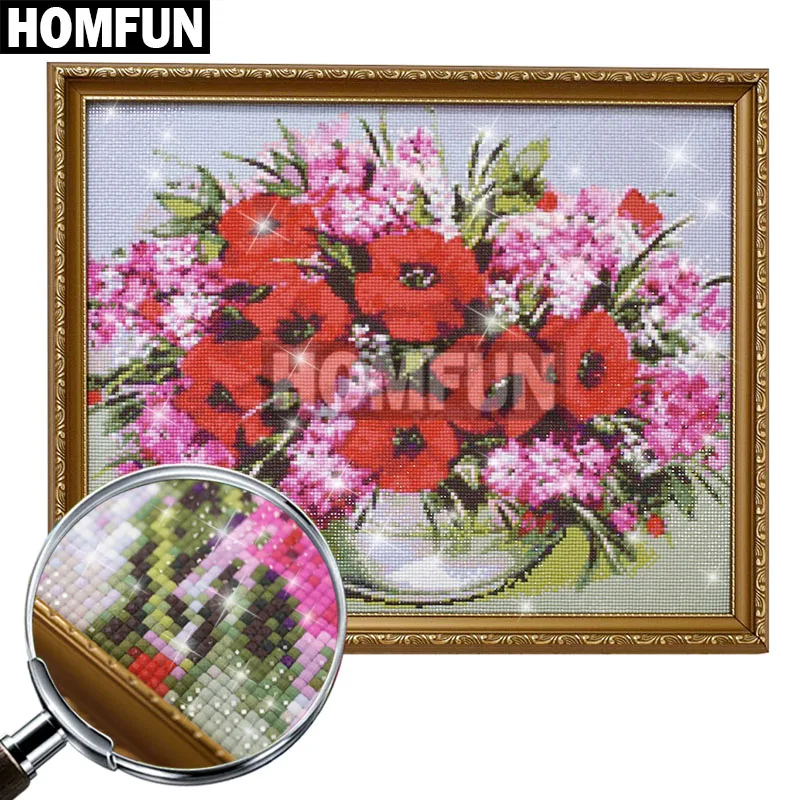The image depicts a vibrant and detailed stitched artwork housed in a decorative coppery frame with a wavy design. At the center of the frame, the craft features a bouquet of red, pink, and white blooming flowers interspersed with lush greenery, all set against a light gray backdrop. The flowers sit inside a white rounded pot. A magnifying glass placed in front of the image zooms in on a section, highlighting the intricate craftsmanship of the small squares or beads used to create the picture. Overlaying the artwork is a semi-transparent black bar with white lettering that reads "Home Fun," also repeated in the upper left-hand corner in red due to the coloration from the flowers underneath. The image is decorated with sparkling lights along the edges and the flowers, adding a touch of whimsy. White circles are visible in the background, adding to the decorative effect.